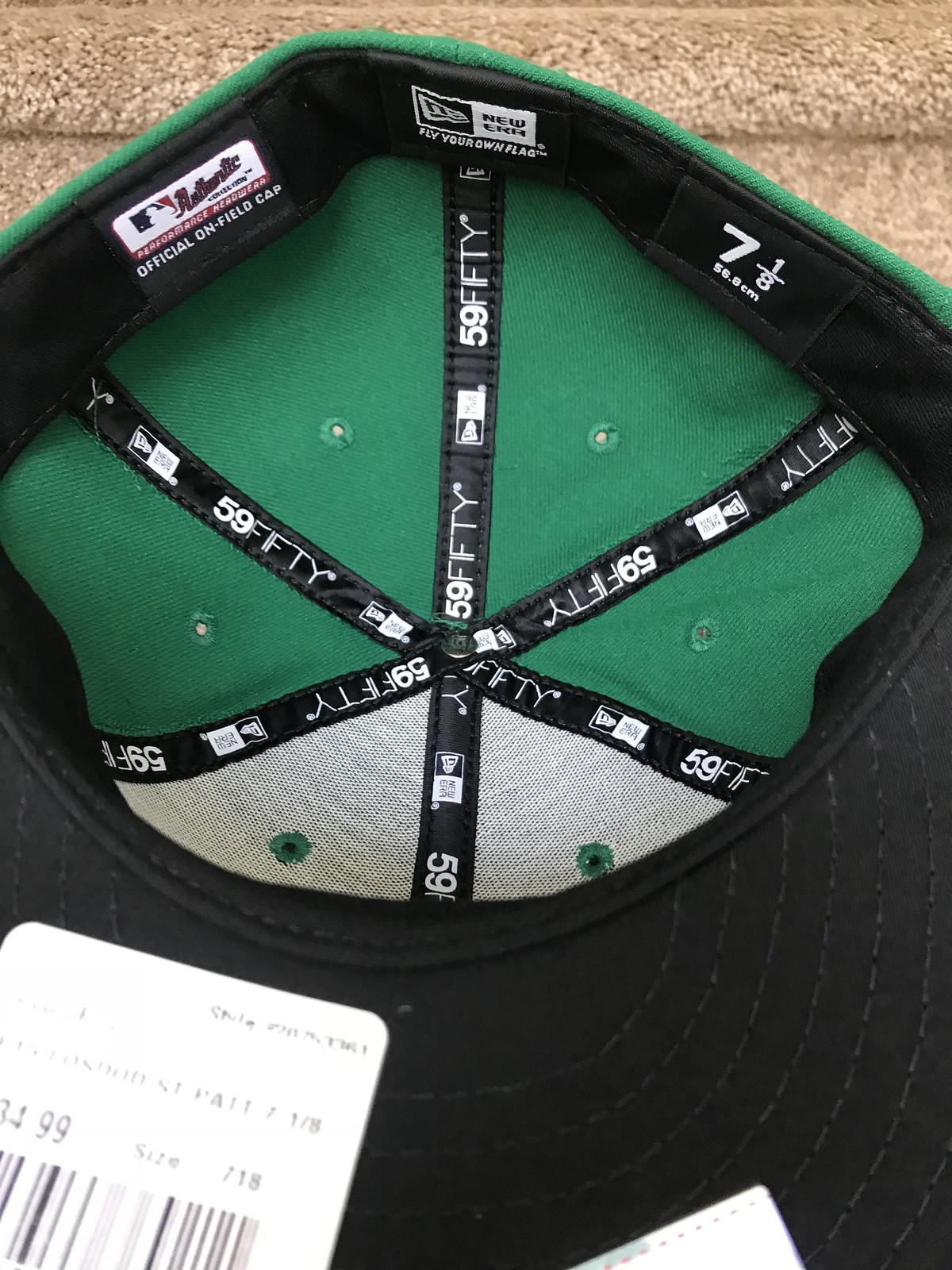This detailed photograph reveals the inside of a baseball cap flipped upside down, offering a top-down view into its inner structure. The entire inner rim of the cap, which sits against your head, is visible and features a black band with distinct white lettering. Notable inscriptions on this black trim band include "official on-field cap," "authentic performance headwear," "fly your own flag," and "New Era." The band also marks the size of the cap as "7 1/8" or "56.8 centimeters."

A central press stud is surrounded by six radial spokes extending outward, with four of the sections between the spokes colored in a vivid clover green and the front two sections in white. The black brim, partially visible and positioned at the bottom of the image, bears a price tag displaying "$34.99" and a partially visible barcode with horizontal black lines. Details such as a mesh-like white fabric are seen toward the front interior, and six small breathing holes punctuate the cap's surface.

The cap's iconic "5950" logo is sewn along the radial spokes and its peak features a design of concentric half semicircles with a concave orientation pointing downward, presented in a slightly overexposed and blurred manner. Additionally, the photograph's background surface appears to be an off-white carpet, possibly placed on stairs.